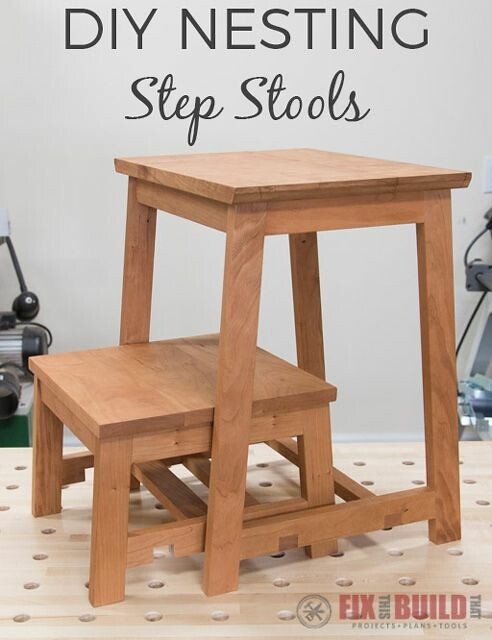This advertisement showcases plans for DIY Nesting Step Stools, prominently displayed at the top in bold black letters against a white wall. Central to the image are two wooden footstools with a maple-colored, flat stain finish. The taller stool stands about two feet high, while the smaller stool is approximately half that height. They feature notched bottom slats, allowing the smaller stool to nest securely within the taller one. These stools are set against a pale wooden board, possibly a pegboard, that is filled with evenly spaced circular holes—suggesting a crafting or woodworking context. To the bottom right, in red lettering, it reads "Fix This, Build That," accompanied by a circular logo with several tools, and below that in dark lettering, it states "Projects, Plans, Tools." Flanking the stools, partially visible, are black and steel machinery pieces, likely tools used in woodworking or industrial tasks, adding to the DIY theme of the advertisement.